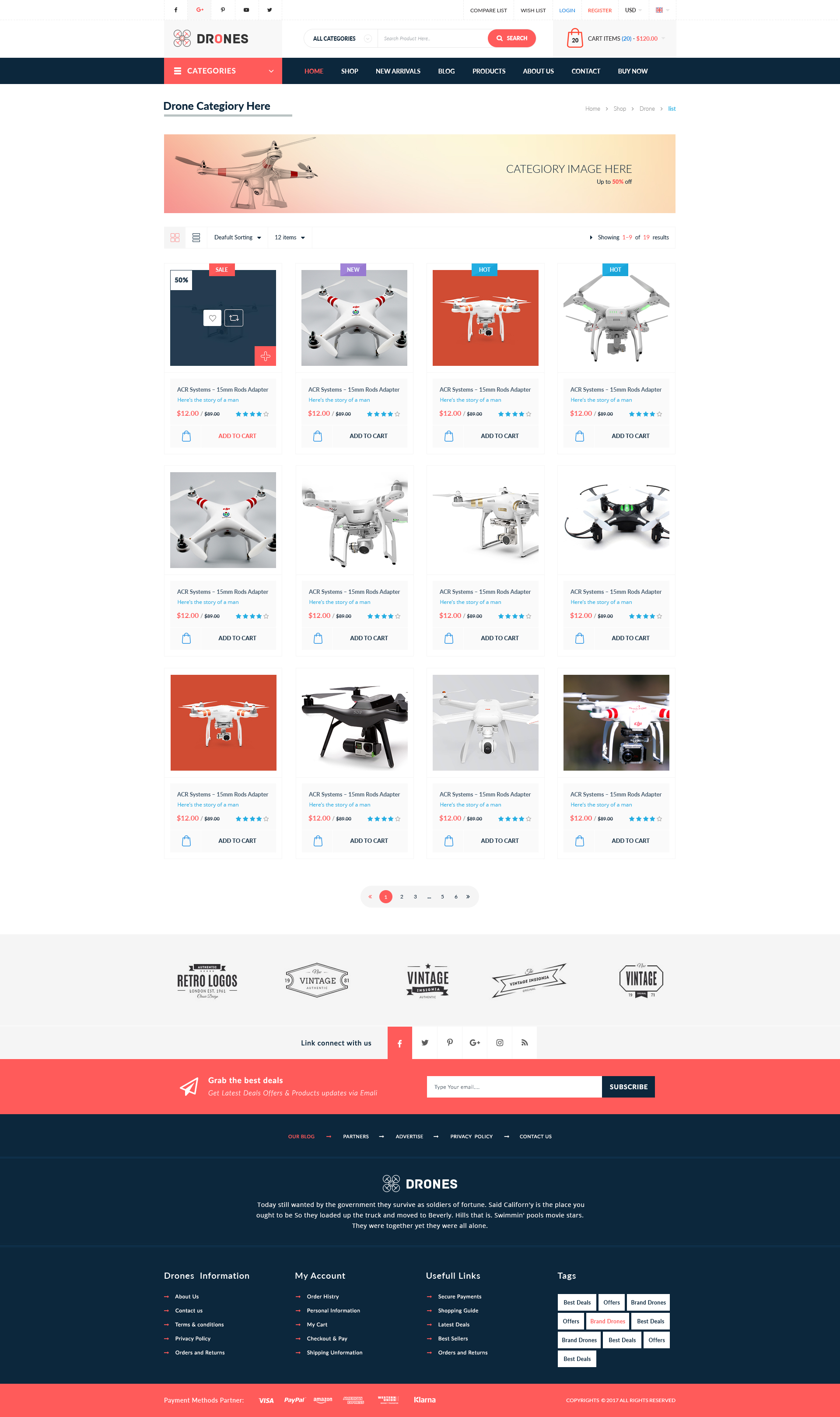This image features a webpage from a drone-selling website. At the top, the logo prominently displays "D-R-O-N-E-S" in black, with the letter "O" being an orange circle. Adjacent to the logo is a design of interconnected circles with X's inside each, set against a white background.

Beneath the logo, navigation options are available, including a search bar, a cart showing $20 worth of items out of $120, a compare list, wish list, login, register, and currency choice (USD). Below, an orange bar with white letters contains categories: Home, Shop, New Arrivals, Blog, Products, About Us, Contact, and Buy Now.

On the right, breadcrumb navigation shows the user's path: Home > Shop > Drone List. An announcement in the category section indicates "Up to 50% off," accompanied by an image of a white drone.

The product listing follows with sorting options, showing 12 items per page. The first four products are white drones labeled "ARC 15 rods adapter," priced at $12 each. There's a mix of sale labels, including "50% Off," "New," and "Hot," though one sale item lacks an image. Each product has an "Add to Cart" option and a four-star rating. The view is set to Page 1.

At the bottom, additional content includes retro and vintage-themed logos. Social media links for Facebook, Twitter, Pinterest, Google, and Instagram are present. A subscription prompt encourages users to enter their email for the latest deals and updates.

Footer sections offer clickable links to various site aspects: Blog, Partners, Advertise, Privacy Policy, and Contact Us. A detailed account management area features options for orders, personal info, cart, checkout, shipping info, and useful links.

The bottommost section highlights secure payment methods like Visa, PayPal, and Amazon, along with obscure logos. The page concludes with a copyright note: "2017, All Rights Reserved."